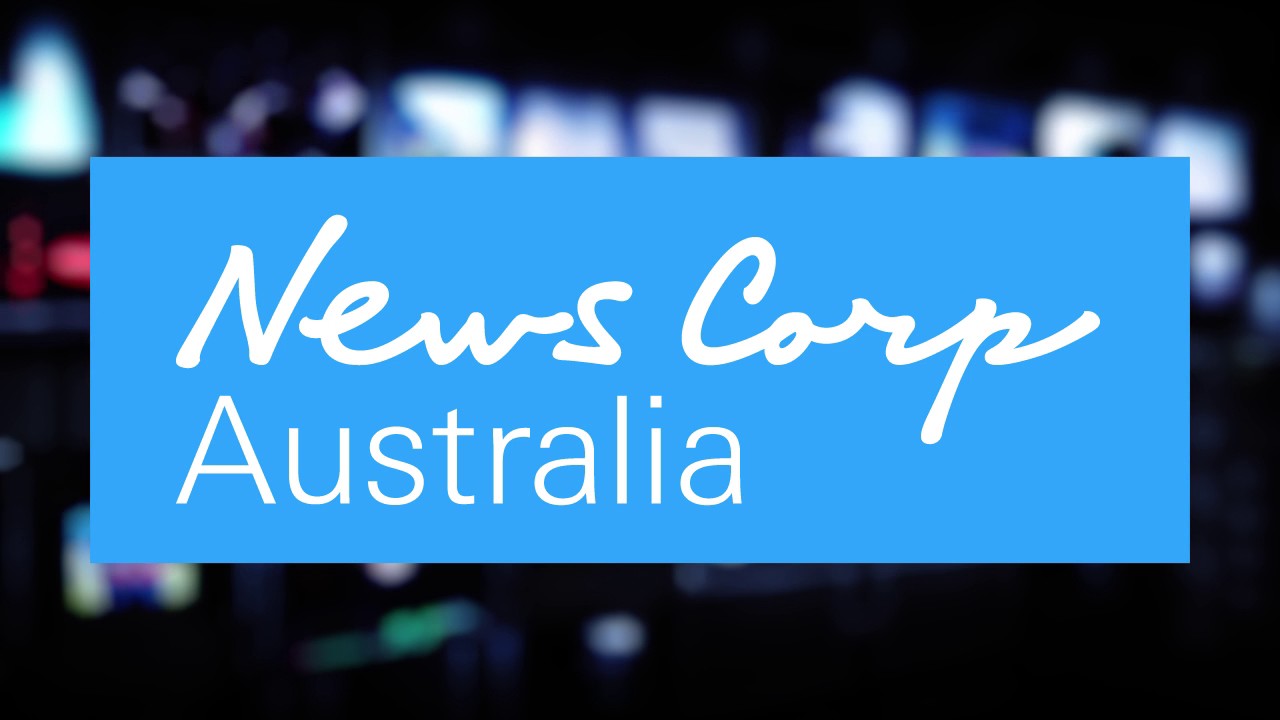The image features a primarily black background around the top and bottom edges, creating a vignette effect. The central focus is a light blue box with the words "News Corp" inscribed in a white, handwritten-style font. Below this, in a more traditional white typeface, the word "Australia" is displayed. Above the blue box, there are several white square shapes that resemble either windows or reflections, contributing to the overall blurred and abstract nature of the background. Notable hints of color include a splash of red on the left side and green mixed with white dots at the bottom left, adding subtle visual diversity to the scene. The blurred effect throughout the image gives it a dreamy and somewhat enigmatic feel.